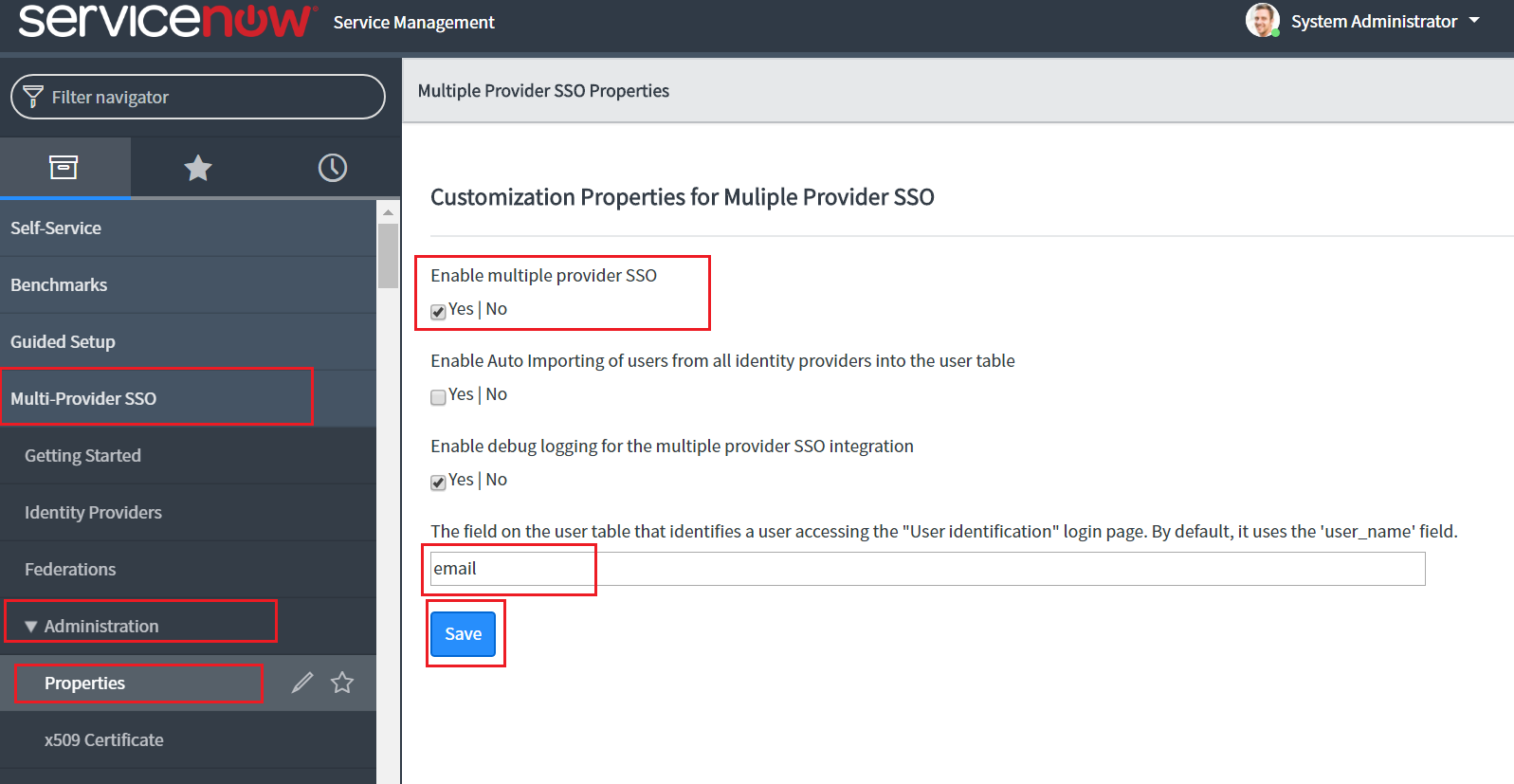The image showcases a webpage with a predominantly black background, featuring various interface elements and text predominantly in white. At the top center, "ServiceNow" is prominently displayed in a mix of white and red text. Below, a black banner with "Service Management" written in white stretches across the page. On the left side, there's a vertical black panel hosting a circular profile photo of a smiling man labeled "System Administrator" with a down arrow for more options.

At the very top of the left panel, a filter navigator button is visible. Adjacent to this panel, there are several navigation buttons, including a star logo in the center and a clock icon on the right. Listed navigation options include "Self-Service," "Benchmarks," "Guided Setup," and "Multi-provider SSO," the latter of which is highlighted in red.

Further detailed options under "Multi-provider SSO" are expanded and include "Getting Started," "Identity Providers," "Federations," and "Administration," with "Administration" further highlighted in red. The "Properties" section is also highlighted in red, indicating active selection or editing. Next to these options, icons for editing (a pencil) and a star button, often used to favorite items, are also visible.

Below the interface list, the term "X-509 Certificate" is displayed. On the right side of the page, detailed information about "Multiple Provider SSO Properties" is provided. This section elaborates on customization properties for multiple provider single sign-on, including an option highlighted in red to "Enable Multiple Provider Single Sign-On."

This descriptively rich image provides a comprehensive view of a system administration interface, highlighting key elements and functionalities in the context of service management with ServiceNow.